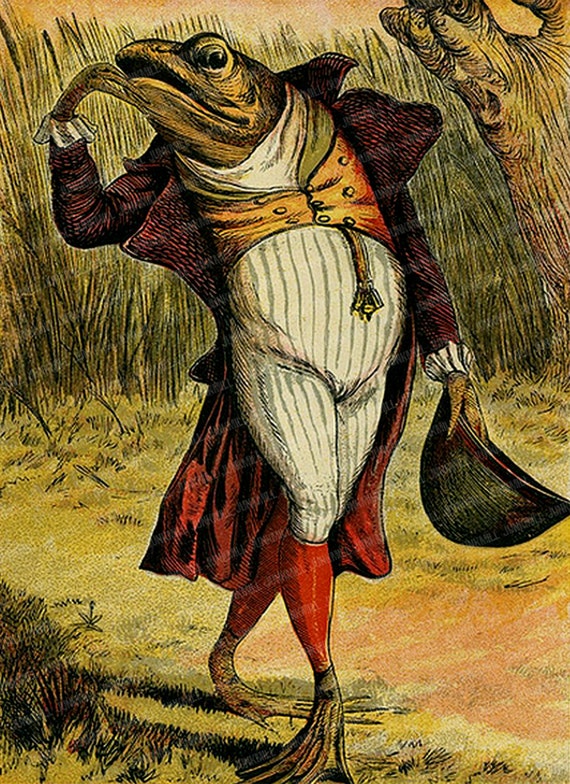The detailed, single descriptive caption for the image could be:

"A vintage color illustration features an anthropomorphized frog, clad in an elaborate 19th-century outfit, walking through a green and yellow grassy woodland. The frog, viewed in portrait orientation, sports an elongated face with a wide, slightly open mouth and bulging eyes that gaze thoughtfully back at the viewer. It wears a dark red overcoat with white lacy sleeves at the cuffs, left open to reveal a gold vest with a green collar, and a white shirt underneath. The frog's extremely high-waisted, gray-striped pants cover its pod belly and reach up to its chest, tucked into red knee socks. It carries a black top hat in its webbed left hand while its right hand is raised pensively to its chin. A white scarf adorns its neck, and a pocket watch hangs from its waistcoat. The background showcases a green and yellow grassy field, with patches of reddish dirt paths and a partially visible tree trunk in the upper right corner, adding depth to the forested scene."